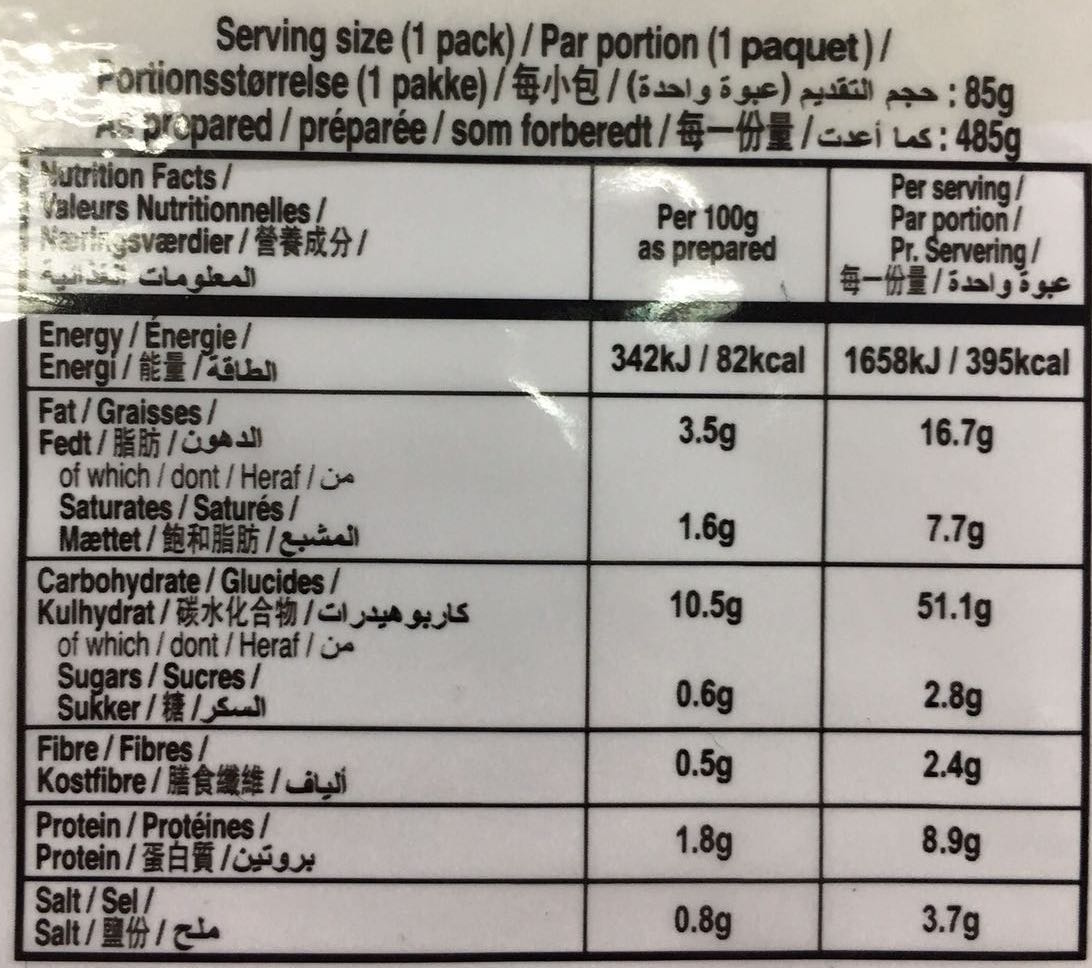This close-up, black-and-white photograph captures the nutrition label on the back of a food package, which appears to be on shiny or possibly laminated paper. The label includes a reflection in the upper left corner. The header at the top indicates the serving size as "1 pack" (par portion, 1 packet) and is presented in multiple languages—at least three, possibly up to five. The nutritional information is organized into three columns: the first column on the left, "per 100 grams" in the center, and "per serving" on the right. The nutrients listed are energy, fat, carbohydrates, fiber, protein, and salt. The center column shows values per 100 grams: 342 kJ/82 kcal, 3.5 grams of fat, 1.6 grams of carbohydrates, 10.5 grams of fiber, 0.6 grams of protein, and 0.08 grams of salt. The far right column details the per serving values: 1658 kJ/395 kcal, 16.7 grams of fat, 7.7 grams of carbohydrates, 51.1 grams of fiber, 2.8 grams of protein, and 3.7 grams of salt.